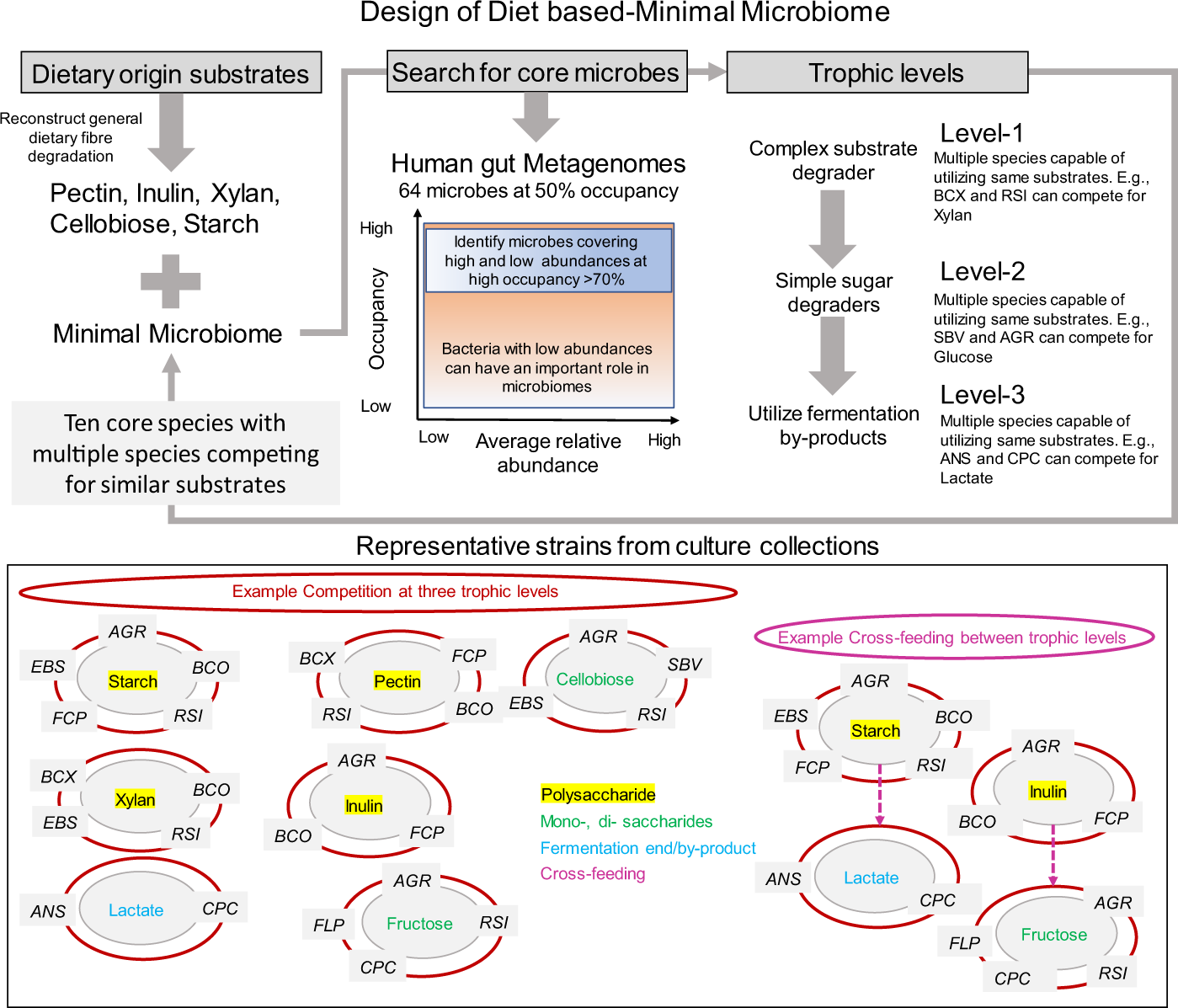The infographic titled "Design of Diet-Based Minimal Microbiome" is divided into two main sections, meticulously detailing the step-by-step process of constructing a minimal microbiome based on dietary substrates. The top section highlights three interconnected subsections:

1. **Dietary Origin Substrates**:
   - Lists dietary fibers like pectin, inulin, xylan, cellobiose, and starch.
   - These substrates are linked to the concept of a minimal microbiome.

2. **Search for Core Microbes**:
   - Focuses on identifying microbes in the human gut metagenomes with 64 microbes occupying 50% frequency.
   - Emphasizes identifying key microbes based on high occupancy (greater than 70%) and low abundance roles in microbiomes.

3. **Trophic Levels**:
   - Explains the trophic structure, detailing three levels where multiple species compete for the same substrates:
     - Level 1: Species competing for xylan (e.g., BCX and RSI).
     - Level 2: Species competing for glucose (e.g., SPV and AGR).
     - Level 3: Species competing for lactate (e.g., ANS and CPC).
   - Indicates that ten core species exist with competition for similar substrates.

An arrow connects the concept of trophic levels back to the dietary origin substrates, forming a feedback loop emphasizing the dynamic interactions within the microbiome.

The bottom section elaborates on:
- **Representative Strains from Culture Collections**:
  - Shows examples of competition at three trophic levels involving starch, pectin, xylan, and inulin.
  - Illustrates cross-feeding between trophic levels, connecting substrates like starch and lactate with various abbreviations representing different strains.

This detailed diagram serves as an educational tool, potentially from a scientific or medical resource, visualizing the complex interactions and roles of different microbes in a diet-based minimal microbiome.